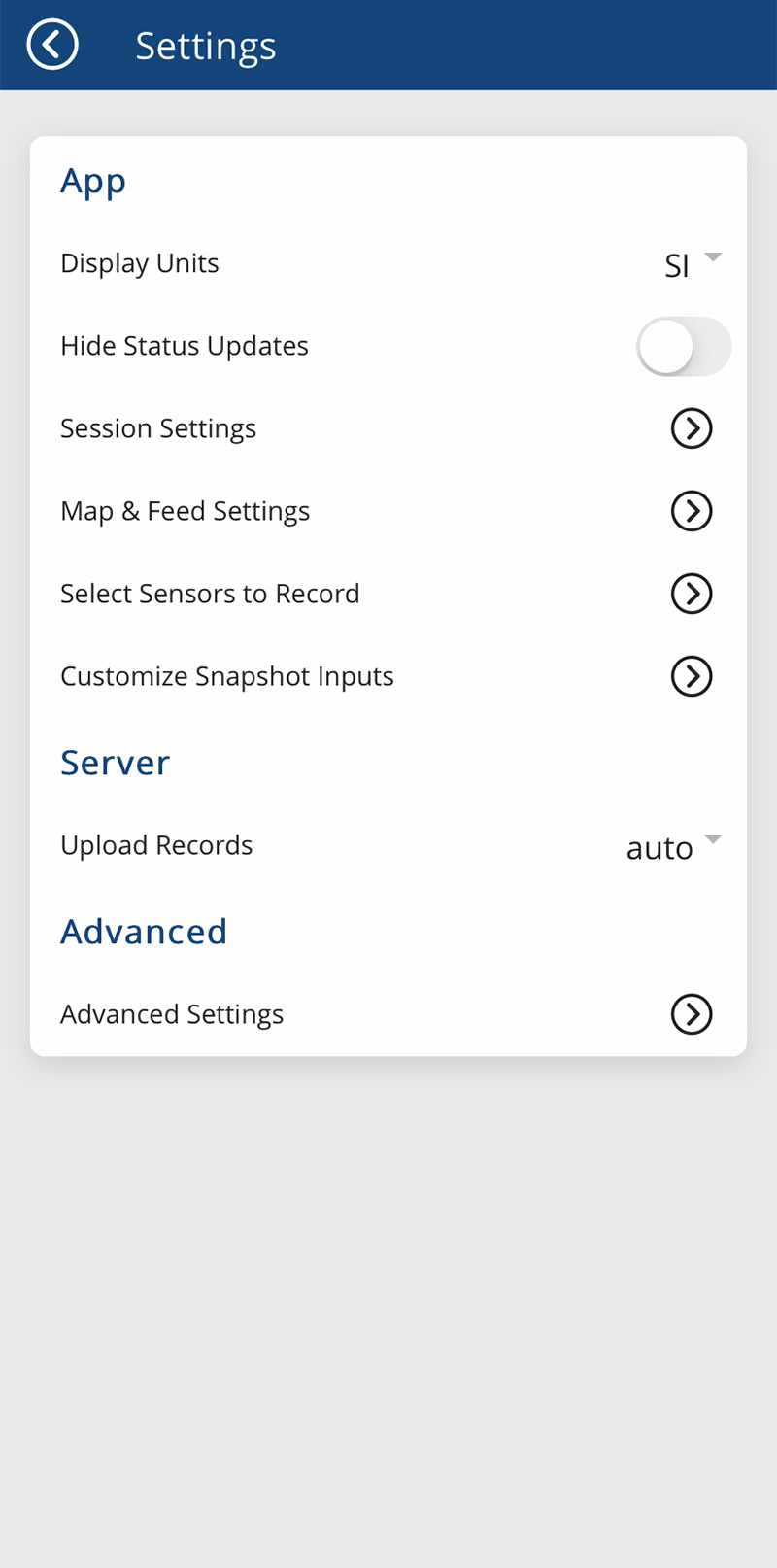Screenshot of App Settings Page:

At the top of the screenshot, there is a dark blue banner labeled "Settings" on the left side. To the left of "Settings," there's an arrow within a circle pointing to the left, indicating a back button. Below this banner, the background of the app is light blue, and it features an overlaid white box containing the primary settings options.

In the top left corner of the white box, "App" is written in blue text. Below "App," there are several categories also highlighted in blue: "Server" and "Advanced." 

Under the "App" category, the following settings are listed:
1. **Display Units**: Positioned on the right side, it displays "SI" with a dropdown box for selecting units.
2. **Hide Status Updates**: A toggle switch that is currently set to off.
3. **Season Settings**: There is an arrow pointing to the right, indicating additional settings can be accessed.
4. **Map and Feed Settings**: Also features an arrow pointing to the right.
5. **Select Sensors to Record**: Accompanied by an arrow pointing to the right.
6. **Customize Snapshot Inputs**: Yet another right-pointing arrow.

Under the "Server" category, the setting "Upload Records" is listed with "Auto" displayed to its right.

Under the "Advanced" category:
1. **Advanced Settings**: Marked with an arrow pointing to the right for further options.

The screenshot captures a structured and user-friendly settings page with various categories and sub-options for customizing the app's performance and user experience.